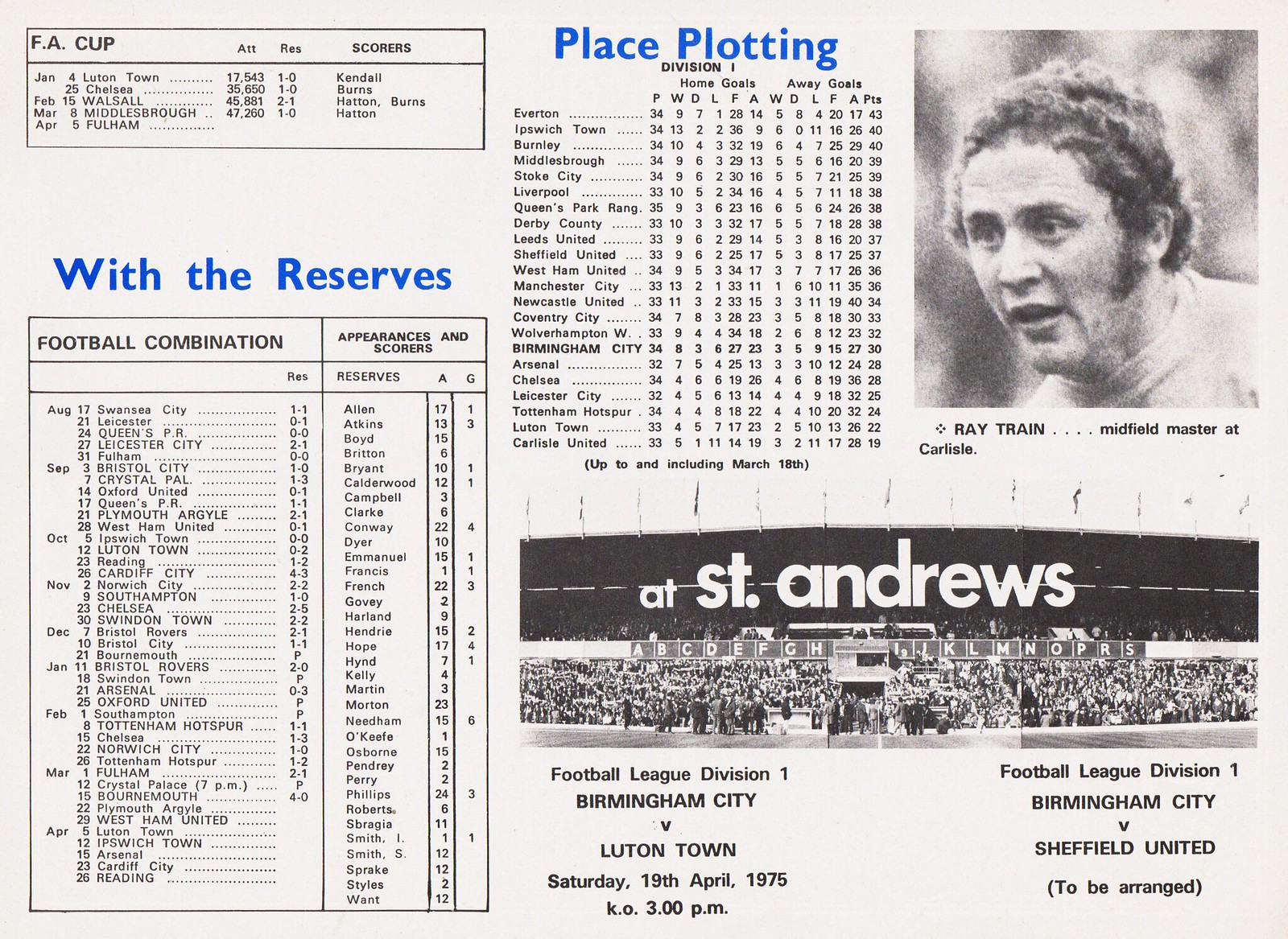The image is a detailed breakdown of soccer standings and player statistics printed on white paper, organized into two primary columns. On the left-hand side, there are two primary sections. The top section features a box in black and white, followed by bold blue lettering that reads "With the Reserves." This section likely details players' appearances and scores in a football combination or reserves format, spanning from August to April. Below this, you'll find another black and white box with more statistical information.

In the middle of the page, another bold blue heading reads "Place Plotting," followed by smaller black text indicating "Division One." This section outlines the home and away goals of various teams, with around 20 teams listed on the left-hand side.

On the right-hand side of the paper, there is a prominent black and white image of a man with curly hair, looking dumbfounded. The caption below the image identifies him as "Ray Train, midfield master at Carlisle." Beneath this, there is another black and white picture, similar in style, capturing a group of people in the stands with white text overlay that reads "at St. Andrew's." Additionally, there is writing indicating a match between Birmingham City and another team, detailing the context of the Football League, Division I.